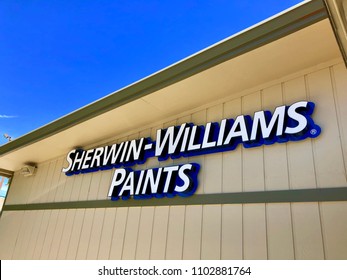A compact landscape image capturing a close-up of a building under a clear blue sky with a wispy white cloud drifting in from the left. The building features white vertical siding with a horizontal gray strip running across it, and the roof is flat, extending out slightly with a mix of gray and white hues. Emblazoned on the side of the building in white letters outlined in blue is the name "Sherwin-Williams," followed by a small copyright symbol. Below the image, there is a text watermark in black, reading "shutterstock.com, 110-288-1764," against a white background.